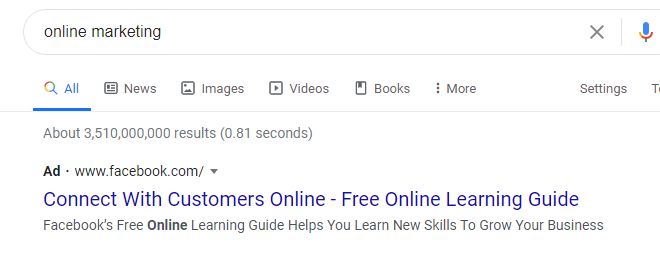The image depicts a screenshot of a Google search bar with the query "online marketing" typed in black text. To the right of this text, there is a gray "X" icon for clearing the search and a microphone icon for voice search. Below the search bar, a rainbow-colored magnifying glass icon is visible, followed by Google’s search buttons. A blue horizontal line underscores the search bar. Adjacent to it, the tabs for different search categories are listed: "All," "News," "Images," "Videos," and "Books." There are also three vertical dots that indicate additional options, along with a "Settings" button. Below these options, a light gray line demarcates the main body of the search results.

The search results section shows a total of about 3,510,000,000 results found in 0.81 seconds. The top result is a paid advertisement promoting Facebook, with a headline suggesting connecting with customers online for free through online learning. No additional results are shown in the visible portion of the screenshot.